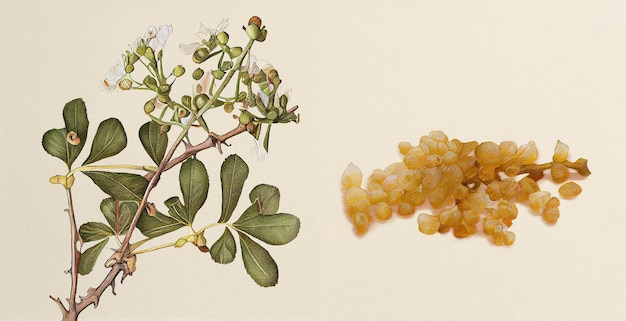This detailed mixed-media artwork features a botanical illustration and a photograph of the medicinal plant, Commiphora wightii (guggul). The cream-colored background sets a neutral tone for the intricate depictions. On the left, a detailed sketch portrays the plant with its woody stem branching into greener offshoots. The lower section of the plant showcases teardrop-shaped green leaves, transitioning upwards to buds and white flowers at the tips. Accompanying this illustration on the right is a photograph of the plant's small, yellowish-brown seeds, carefully arranged on the same beige surface. This combination provides a comprehensive visual study of guggul, highlighting its significant botanical and medicinal characteristics.